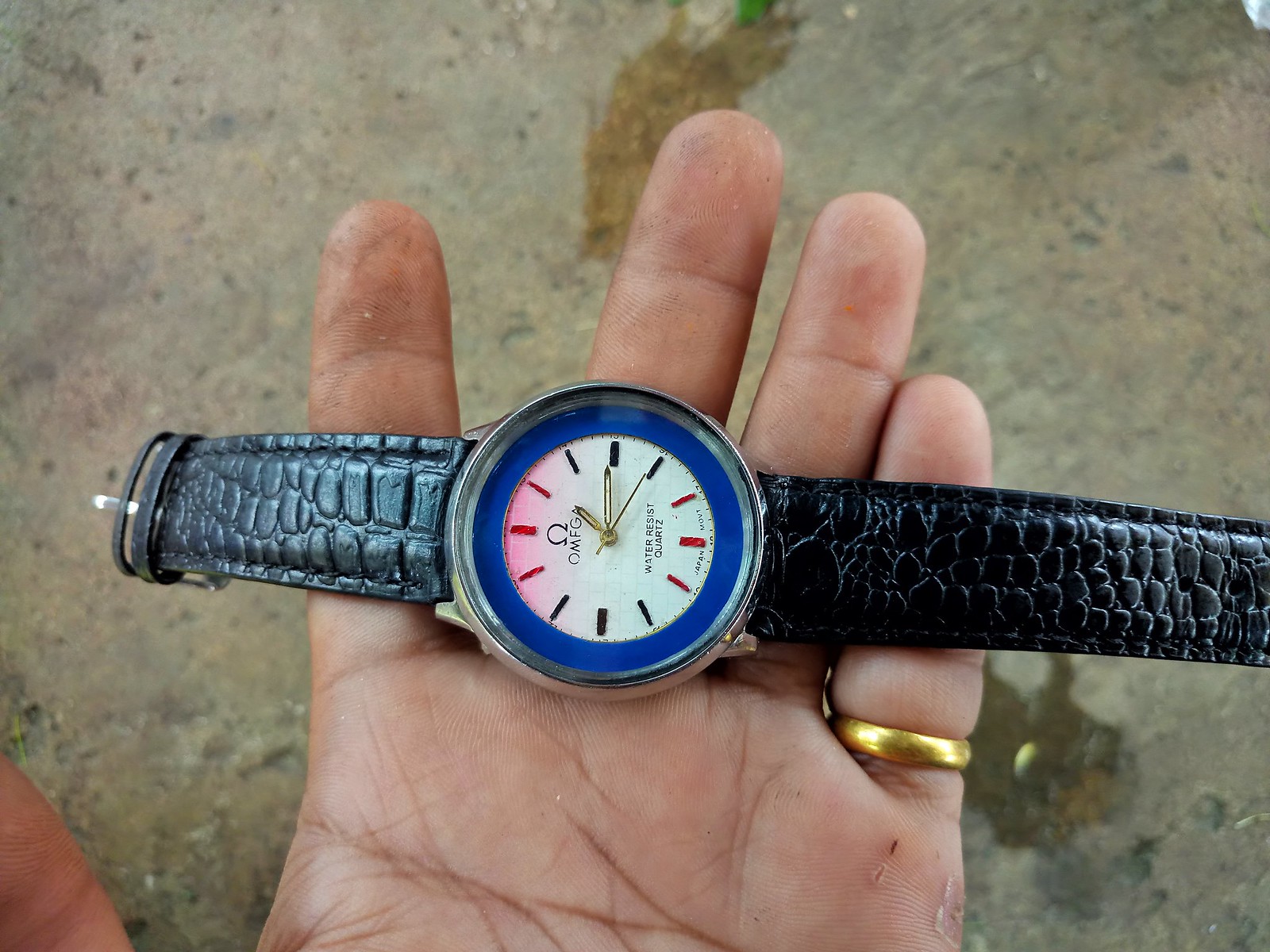In this detailed photograph, a close-up of a person's hand is shown, holding a wristwatch laid flatly across their short and stubby fingertips. The hand belongs to someone likely older, suggested by the appearance of the fingers. The person is wearing a gold ring on their pinky finger. The background is textured ground, primarily brown with greenish-yellow spots.

The wristwatch features a distinctive design with a black leather band that exhibits a cracked, bumpy texture, reminiscent of alligator skin. The watch face is encircled by a silver outer ring, within which lies a blue ring containing the watch's time indicators. Instead of numbers, there are simple line markers denoting the hours. The watch face also includes the label "OMFG" and at the bottom, it has "water-resistant quartz" inscribed.